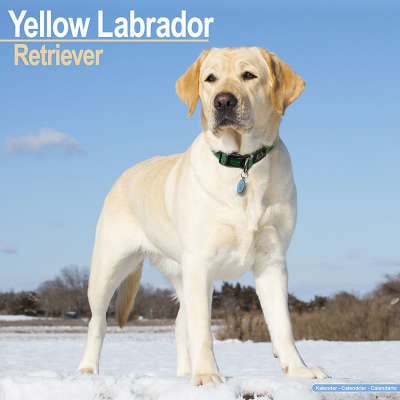This is an image of a yellow Labrador Retriever standing on snowy ground outside. The Labrador has a very light, almost white coat with more tan-colored ears. It is facing the camera, wearing a black collar accented with green and a blue dog tag. The dog's tail points downwards as it stares ahead. The backdrop features brown, leafless trees and bushes, indicating a winter setting. The sky above is a vivid blue with a single white cloud, positioned near where the dog's tail would be. At the top left corner of the image, white text reads "yellow Labrador" and just below it in yellow text, "Retriever." In the bottom right, there's a blue strip with blurred white text on it.